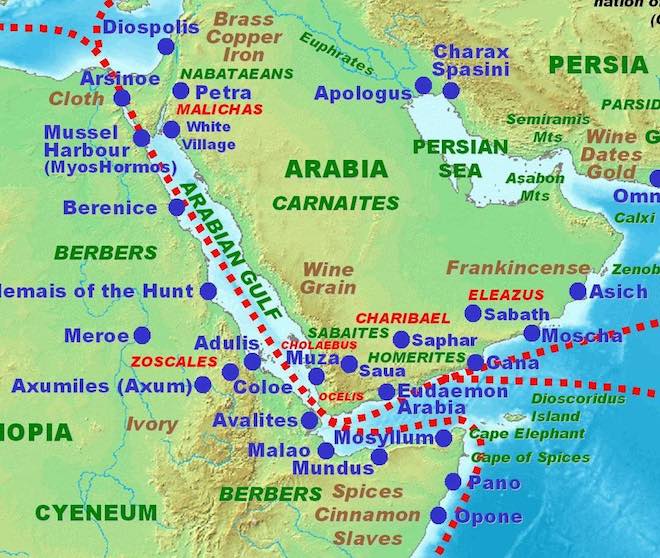This square-shaped, cartoon-style map presents an historical view of the Middle East and parts of northeastern Africa, replete with older nomenclatures such as Arabia, Persia, and Berbers. The land masses are predominantly green with orangish areas marking mountainous regions, and the surrounding waters are illustrated in shades of blue. Key locations and their notable exports are highlighted in different colors: regions are marked with identifiers like frankincense, wine, and grain in Arabia; spices, cinnamon, and slaves along the African coast; and brass, copper, iron, and cloth near Israel. Additionally, there are numerous blue dots scattered across the map, signifying ancient cities such as Petra, Apologos, and Meroe. Red dotted lines traverse from the Mediterranean across the Arabian Gulf, denoting historical trade routes. Furthermore, the map is visually enriched with different colored text to denote various geographic and economic details, providing a vibrant and informative depiction of the area's historical trade networks.